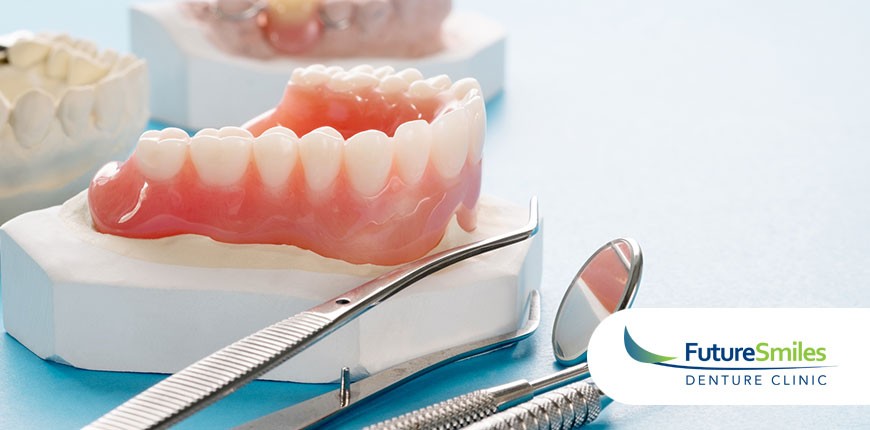The advertisement for "Future Smiles Denture Clinic" features a detailed and vivid image set against a light blue background. At the forefront, there's a clear view of a lower gum line and row of immaculate white teeth attached to a pristine white surface. The gums appear healthy and pink. To the left of this primary set of dentures is a plaster impression of teeth, adding a sense of the clinical process involved in denture creation. Another set of dentures can be seen slightly blurred in the background, highlighting depth and focus in the image. Positioned on the lower right side of the image are three dental tools, including a pair of forceps, a dental mirror, and a third instrument partially obscured by the clinic's logo. The clinic's logo is set within a long oval featuring the words "Future Smiles" in blue and lime green respectively, accented by a half-moon design in matching colors. A black line underscores the name "Future Smiles," with "Denture Clinic" written in blue beneath it on a white background. The overall impression is one of professional care and meticulous attention to dental health, set in a serene and clean aesthetic.